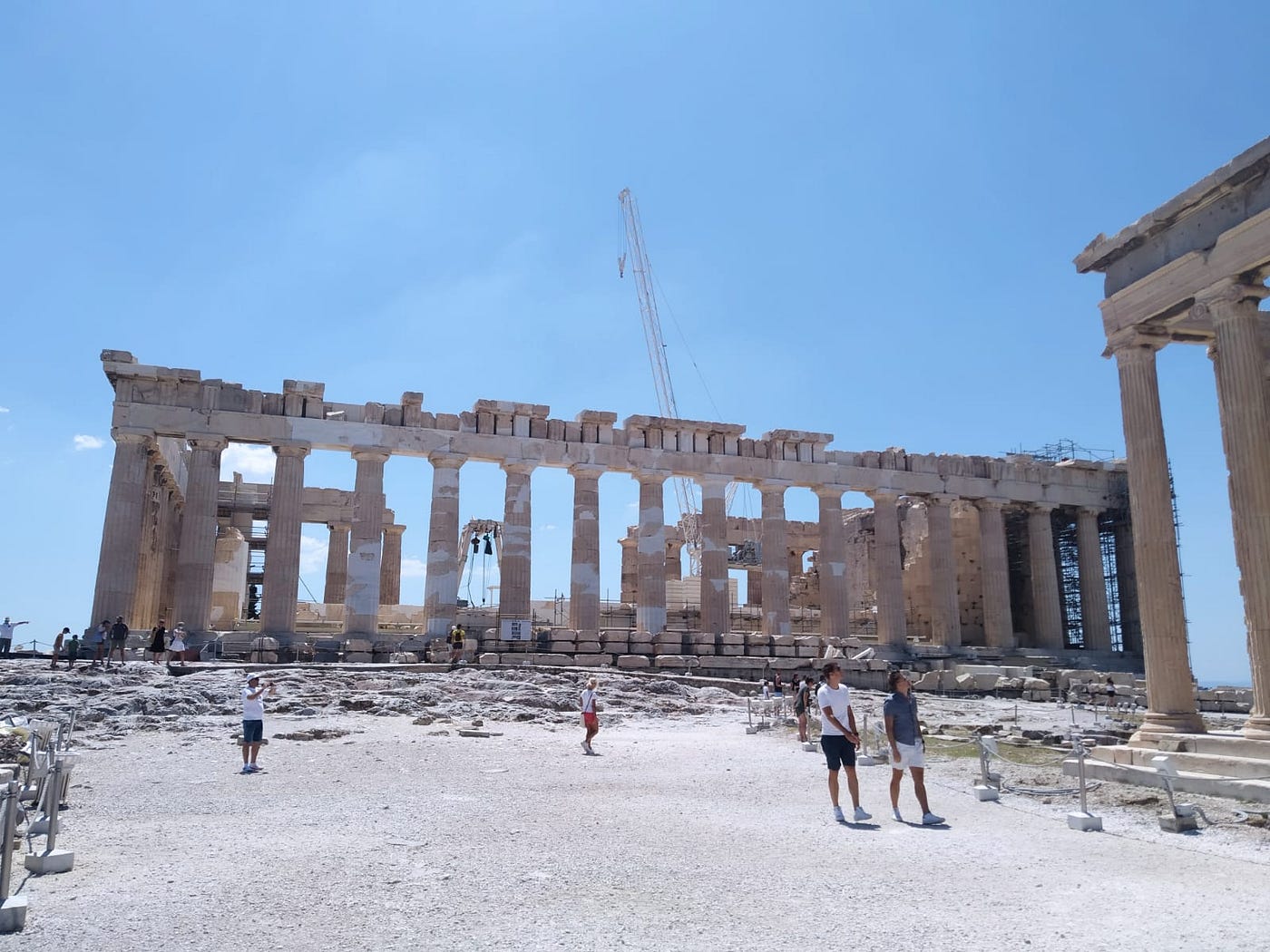This image captures the enduring majesty of ancient Greek ruins under a brilliant clear blue sky, where a multitude of weathered support columns stand as stoic sentinels of history. The scene is animated by tourists strolling on a dirt-covered path, roped off by chain link fences to guide their footsteps and protect the site. Amid the backdrop, a crane looms, signaling ongoing restoration efforts to preserve the deteriorating structure. To the right, portions of the image show areas strewn with rubble, hinting at past collapses. The sun casts sharp shadows directly below the visitors, emphasizing the midday timing of the photo, as they pause to absorb and photograph the historical significance around them. In the background, more visitors are visible, further exploring the expansive remnants of a once-grand architectural marvel.